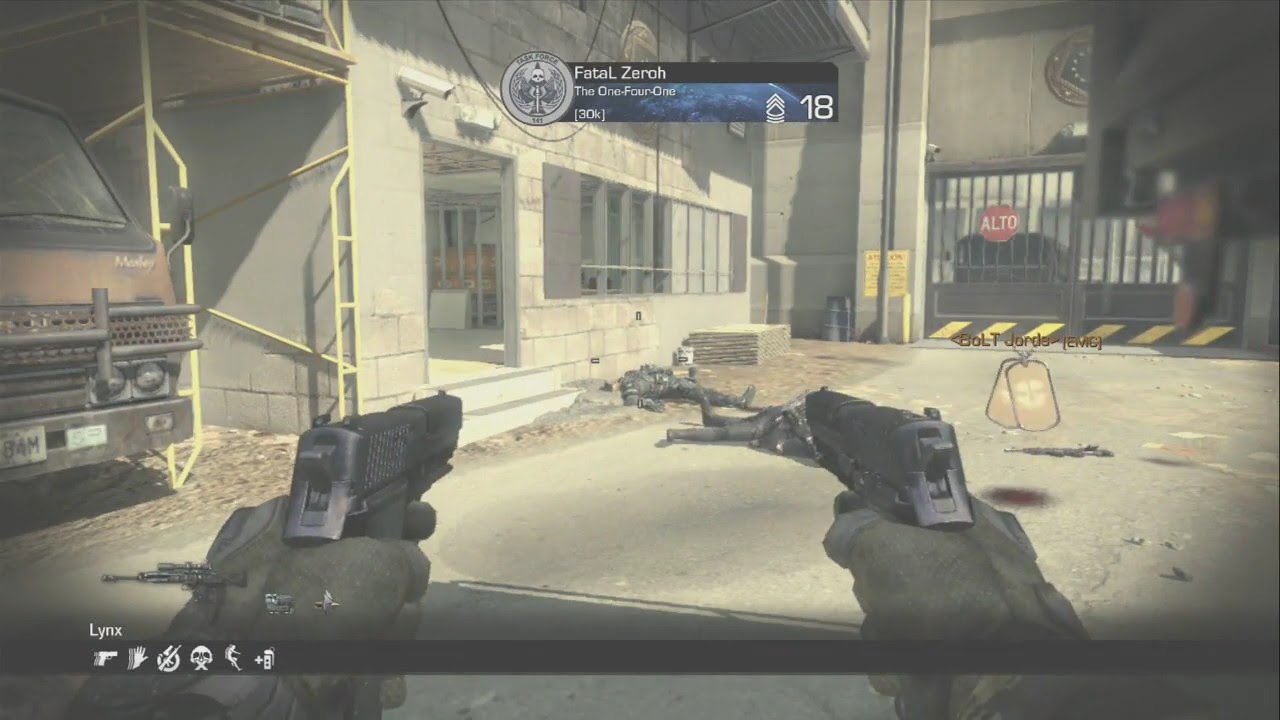This image captures a moment from a first-person shooter video game, resembling titles like Call of Duty or Counter-Strike. At the bottom of the image, the character's hands are extended in a first-person view, each holding a pistol. A thin, black horizontal bar spans the width of the screen, displaying the word "links" on the left, along with icons of a gun, a skull and crossbones, and various other unidentifiable symbols. Above this bar, notifications read "Fatal 0," "the 141," "30k," and "rank 18." 

In the main part of the image, the scene appears to take place in an industrial or construction zone. On the left, a partially visible truck is parked in a bay. There are two downed players or bodies on the ground, with floating dog tags bearing usernames above them. A wall with windows stands to the right, and further right, a stone wall leads to some gates, possibly opening to another building. Cement covers the ground, with a black base and yellow stripes at the bottom of the frame. The environment features dull gray, yellow, silver, red, brown, black, and blue colors. Text elements such as "fatal zero," "links," "alto," and "bolt jords" are part of the game's heads-up display (HUD), which also includes various icons in the bottom left corner.